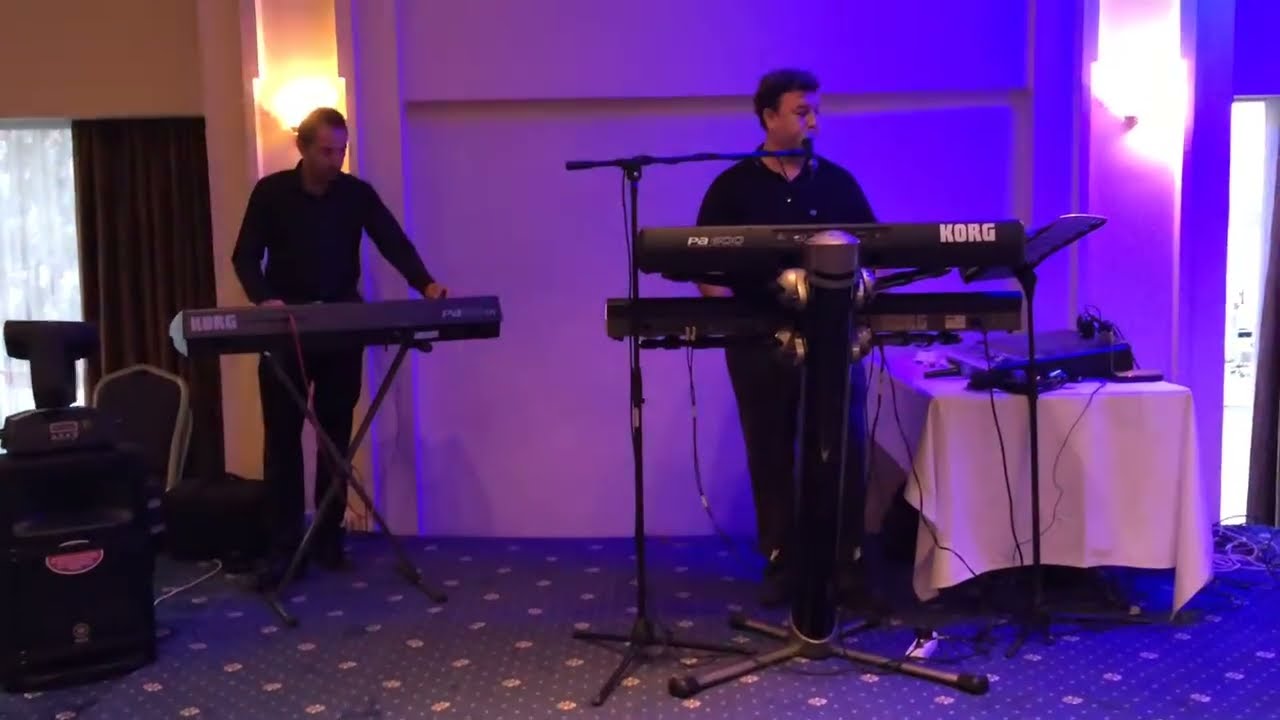In a dimly lit hotel conference room, two musicians stand behind Korg keyboards, bathed in a mix of blue-purple and yellow light. The musician on the left, dressed in all black with a long-sleeve shirt, plays a single keyboard. The brand "KORG" is visible on the left side of his instrument. The musician on the right, also dressed in all black, operates two keyboards and speaks into a microphone attached to a stand positioned at face level. To his right, a table draped in a white tablecloth holds an electronic device, likely a mixing board. The room features patterned carpet and is further illuminated by two sconce lights and possibly a window to the left, suggesting daylight outside.